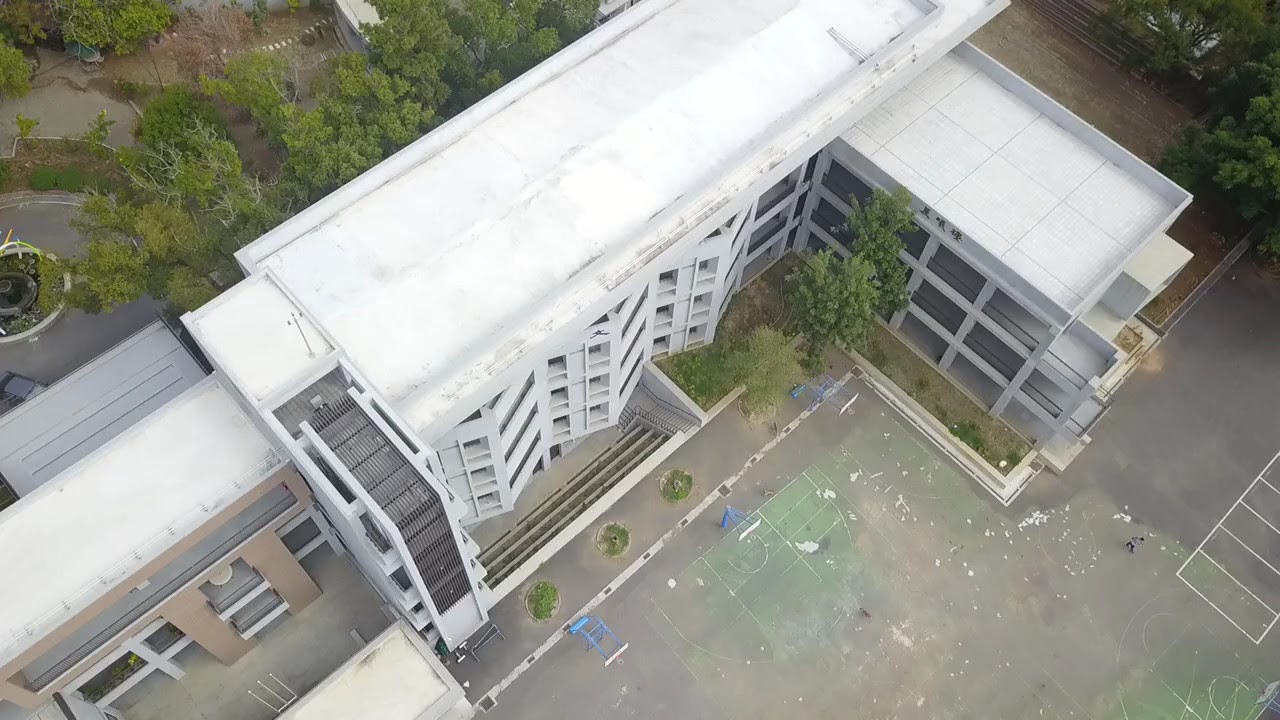This aerial image captures a uniquely shaped, wide, and four-story building centered prominently in the frame. The structure features a combination of flat and curved sections, creating a notable front where a rectangular extension with protruding square windows stands out. The building’s façade is predominantly white, contrasting with a smaller brown annex visible on the left side and a cement-colored annex, likely a parking garage, on the right side. The rooftop appears flat and white, while the surrounding area is vibrant with greenery, including bright green trees behind and around the building, contributing to a well-maintained, garden-like atmosphere. In the bottom right corner, there's a parking lot adjacent to bushes and an exterior concrete area. A rec room is also hinted to exist near the structure. Additionally, there seems to be some construction-related debris scattered in the middle portion of the image, complementing the visible concrete and possible fountain in the back left. Overall, the photograph captures the outdoor setting in the middle of the day with an intricate depiction of the building's surroundings and details.